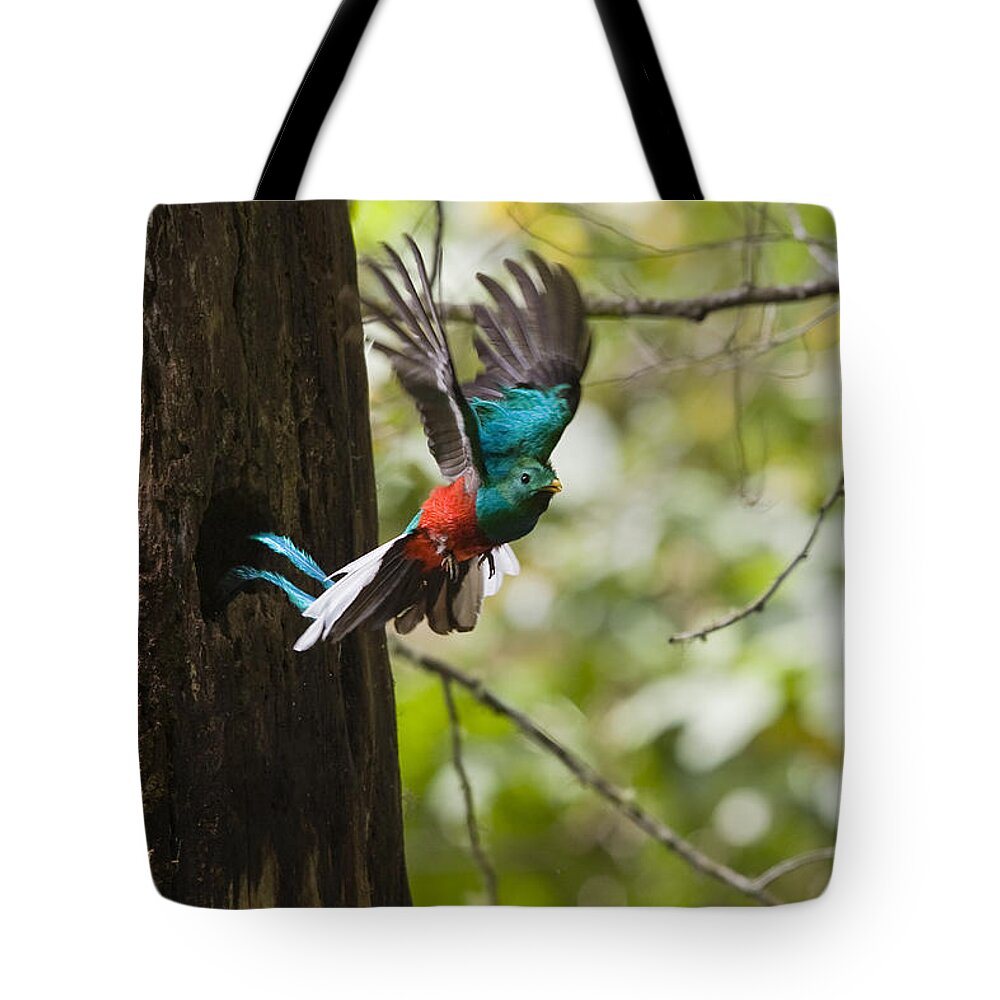The image is of a colorful tote bag with black straps, featuring a highly detailed and vibrant stock photo of a bird. The bird, captured in mid-flight as it exits a hole in a tree, displays a striking array of colors, including a greenish-teal head and wings, dark gray or black outer feathers, and a vivid red body. The bird’s tail is fanned out, showcasing white feathers along with long teal feathers trailing down past the tail. The background consists of blurred branches and tree foliage with some faded green and white leaves, possibly illuminated by sunlight filtering through. The bird’s side profile is prominent, highlighting its small black eye and tiny yellow beak, making it the focal point of the image.